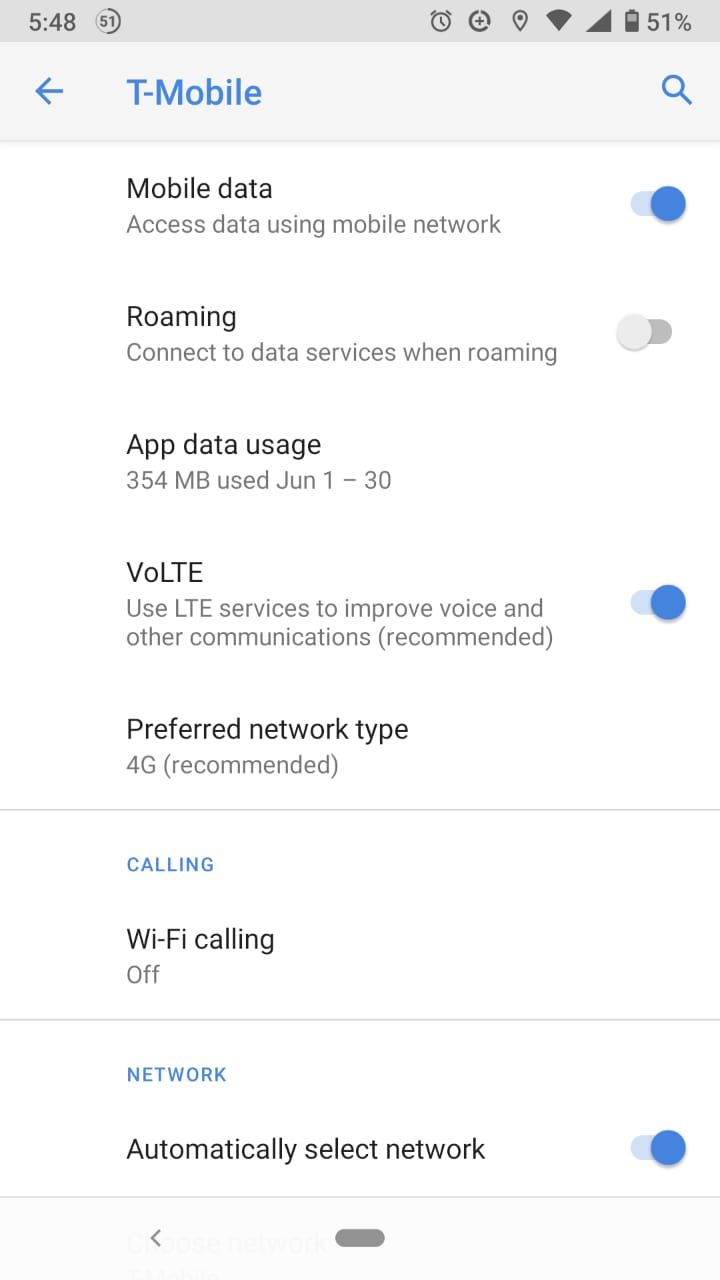The image features a detailed screenshot of an individual's T-Mobile settings on their smartphone. 

At the top of the image, the time is displayed as 5:48, indicating the current time. The phone's signal strength is strong, and the battery is at 51% capacity. Several icons are also visible in this area, including one that resembles an alarm clock and another that could be a search function.

Under the settings, the "Mobile Data" option is highlighted, indicating that the phone can access data through the mobile network, and this feature is enabled. "Roaming," which allows the device to connect to data services while roaming, is disabled. 

The section labeled "App Data Usage" provides information on data consumption from June 1st to June 30th, totaling 354 megabytes. 

Next, "VOLTE" is enabled, showcasing the use of LTE services to enhance voice and communication quality, a recommended setting. The preferred network type is set to "4G." 

"Wi-Fi Calling" is presently turned off, and the "Network" setting is configured to automatically select the best available network, which is enabled.

Overall, this smartphone setup indicates a well-configured device, optimized for both data usage and network performance, with a balance of necessary functionalities enabled.